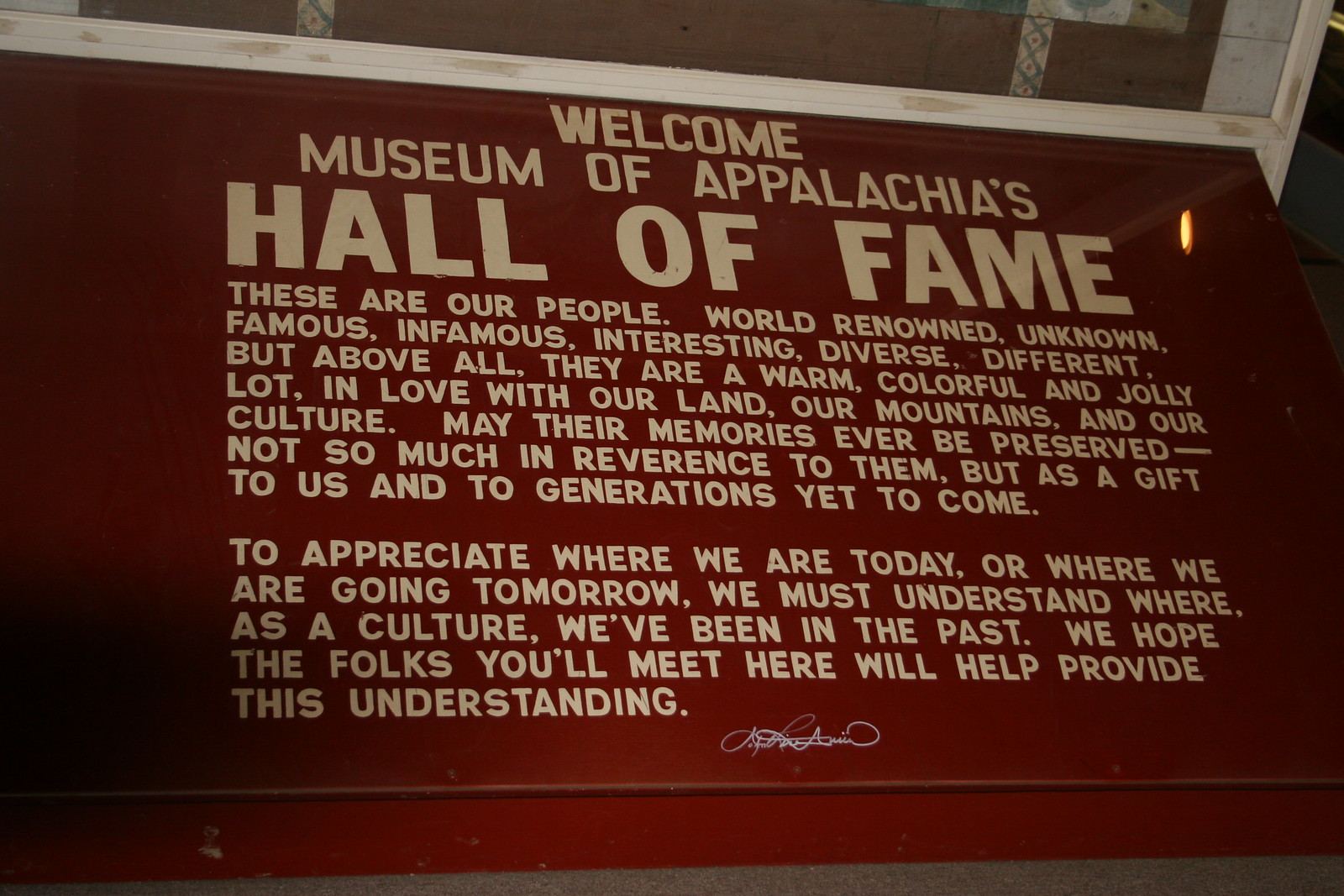The image is a color photograph in landscape orientation featuring a large placard positioned close to the ceiling on a reddish-brown wall, possibly above a window or doorway bordered in white. The placard, written in white text, reads: "Welcome to the Museum of Appalachia's Hall of Fame." The phrase "Hall of Fame" is prominently displayed in very large letters. The text continues, describing the people it honors as "world-renowned, unknown, famous, infamous, interesting, diverse, different," but above all, "warm, colorful, and a jolly lot in love with our land, our mountains, and our culture." The inscription emphasizes the importance of preserving their memories not just in reverence to them, but as a gift to future generations, to help understand where the culture has been in the past and to appreciate where it is heading. The detailed, heartfelt message reflects on the connection to the land and the importance of cultural heritage. There is an illegible signature in white at the bottom of the placard. The overall style captures a realistic and representative depiction of the message.